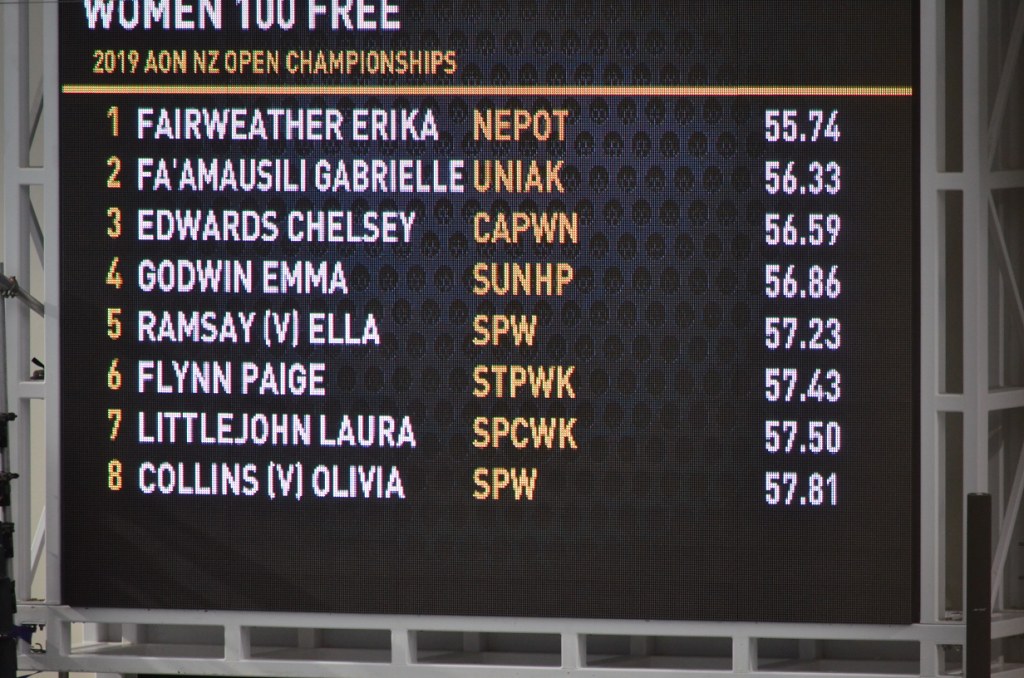The image portrays a scoreboard from the 2019 Aon New Zealand Open Championships, specifically for the Women's 100-meter freestyle event. The board features a simple design with a black background, and text displayed in white and orange lettering. Supported by a gray material, the scoreboard lists the top eight swimmers along with their times, which range from 55.74 seconds to 57.81 seconds. The leaderboard is headed by Erica Fairweather with a time of 55.74 seconds, followed by Gabrielle Moss-Lily, Chelsea Edwards, Emma Godwin, Ella Ramsay, Paige Flynn, Laura Littlejohn, and Olivia Collins. The clean and straightforward layout ensures clear visibility of the results.